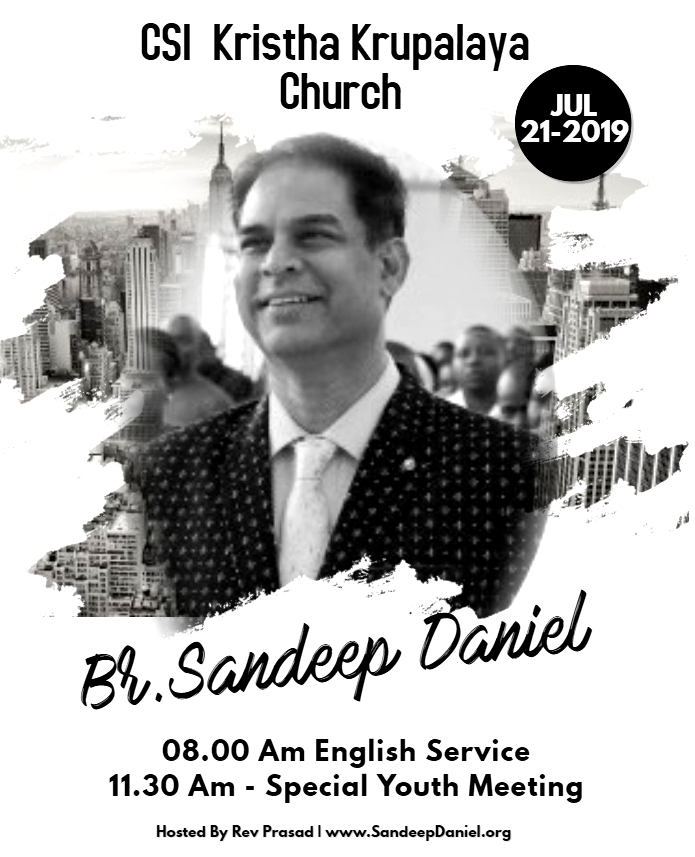This black-and-white promotional flyer for CSI Krista Krupalaya Church prominently features an image of the pastor, Reverend Sandeep Daniel, who is dressed in a dotted suit, a tie, and a white dress shirt. He is positioned in the center of the flyer, looking to the left. People can be seen in the background, along with a high-angle view of city skyscrapers, creating a collage effect on both the left and right sides. At the top of the flyer, bold black text reads "CSI Krista Krupalaya Church." On the right side, a black circle contains the date "JUL 21, 2019" in white text. Below the pastor’s image, additional details are provided: "8:00 a.m. English service, 11:30 a.m. Special youth meeting, hosted by Reverend Prasad." The web address "www.sandeepdaniel.org" is also mentioned for further information. The flyer serves as an advertisement for church services scheduled for July 21, 2019.